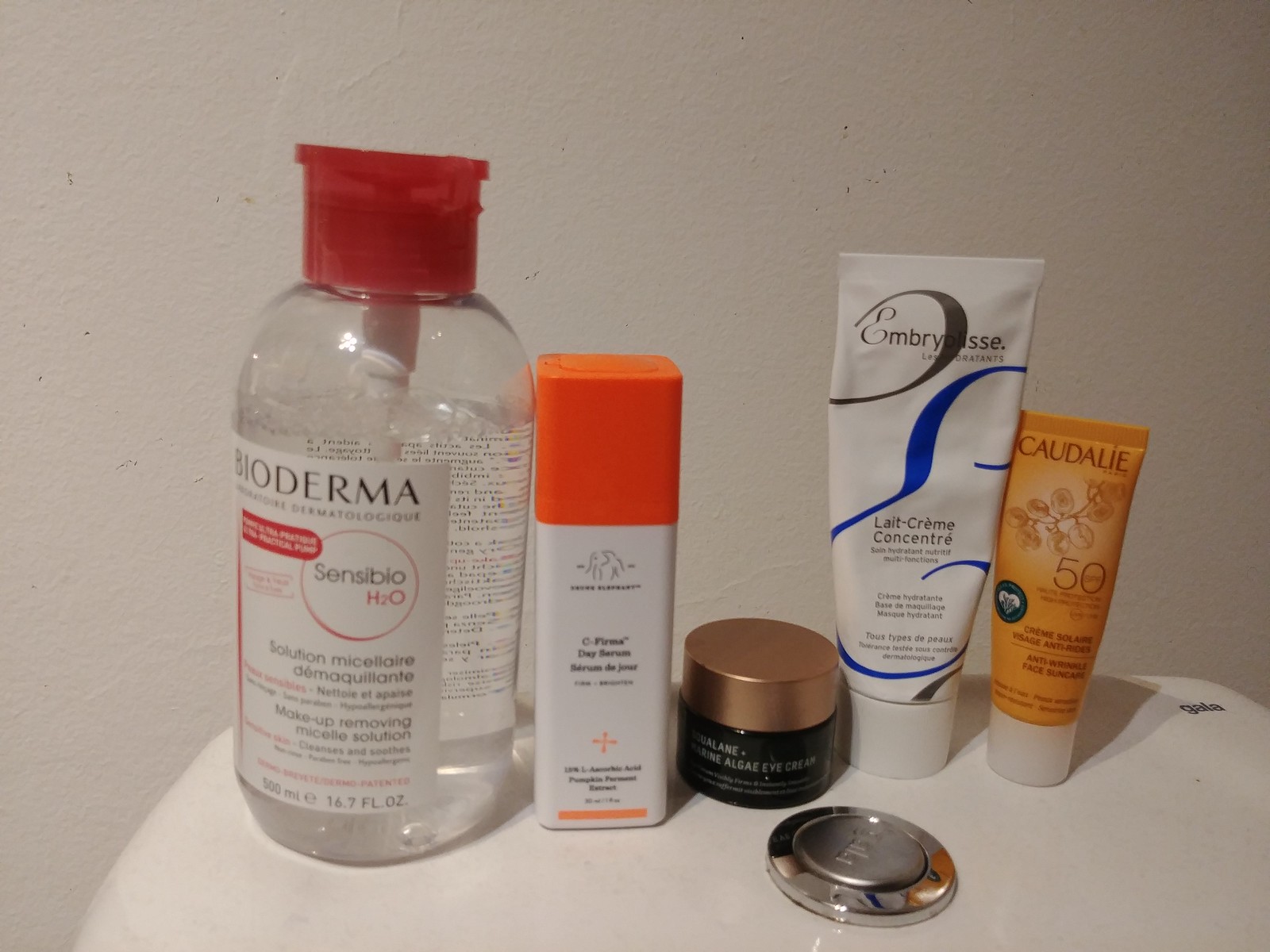The image showcases a collection of five facial skincare products arranged on a porcelain surface, likely the top of a toilet tank, characterized by a white finish with a silver button at the bottom. The background features a plain white wall. 

From left to right, the products are as follows:

1. **Bioderma Sensibio H2O:** This is a clear bottle with a red cap, prominently featuring its logo within a red circle.
  
2. **Unknown Brand:** Next is a product with an orange cap and a white neck. The writing is too small to decipher.
   
3. **Algenist Complete Eye Renewal Balm:** The smallest in size, this is housed in a black jar with a bronze-colored lid, and indicates it is an algae-based eye cream.

4. **Embryolisse Lait-Crème Concentré:** This product is a white tube, with the brand name "Embryolisse" and the product name "Lait-Crème Concentré" written in French.

5. **Caudalie SPF 50:** The final item is an orange bottle labeled "Caudalie," with a reference to an SPF value of 50, suggesting it is a sunscreen product.

The clean and minimalist setup highlights these skincare items against the stark white background, emphasizing their design and packaging.